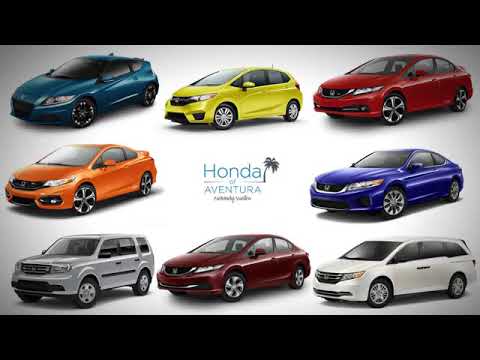This full-color digital advertisement for Honda of Aventura showcases their range of vehicles in a horizontally rectangular layout. The image features a horizontal black stripe at the top and bottom, with a central white background highlighting the dealership's name in blue lettering. Below the text, a right-tilting palm tree logo adds a touch of local flair. Surrounding the central logo are eight distinct photographs of different Honda vehicles, each meticulously presented to exhibit the variety available at the dealership. The advertised cars, positioned around the central logo like a clock face, include a yellow hatchback at 12 o’clock, a red four-door sedan at 1 o’clock, a blue two-door hatchback at 3 o’clock, a white passenger van at 5 o’clock, a burgundy four-door sedan at 6 o’clock, a gray SUV at 7 o’clock, an orange coupe with a spoiler at 9 o’clock, and another blue hatchback at 10 o’clock. This visual arrangement, combined with the advertisement’s photographic and graphic design elements, effectively highlights the diverse array of Honda vehicles available for purchase.